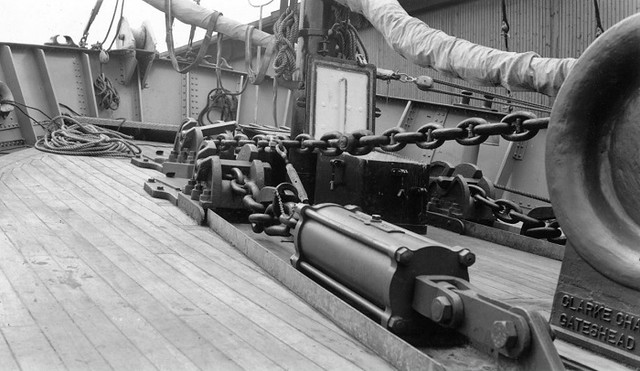This black and white photograph captures a dramatic scene on the deck of a large ship. The overcast sky looms in the background, adding to the moody atmosphere. Prominently featured is a massive anchor chain, heavy-duty and seemingly in motion, slipping backward across the wooden planks of the deck, which appear uneven, giving the impression of the ship being tilted. The chain feeds into a metal apparatus, likely some type of pump, and wraps around another metal component marked with the partially readable label "Clark O-H-A Gatehead." The ship's deck is lined with metal railings fastened with rivets, interspersed with ropes, pulleys, and possibly folded sails, indicative of the ship's sailing equipment. Masts extend upwards, with various wires and ropes hanging, contributing to the intricate maritime setup. The angled perspective of the photograph evokes a sense of urgency and instability, reminiscent of the chaotic moments on a ship in distress.